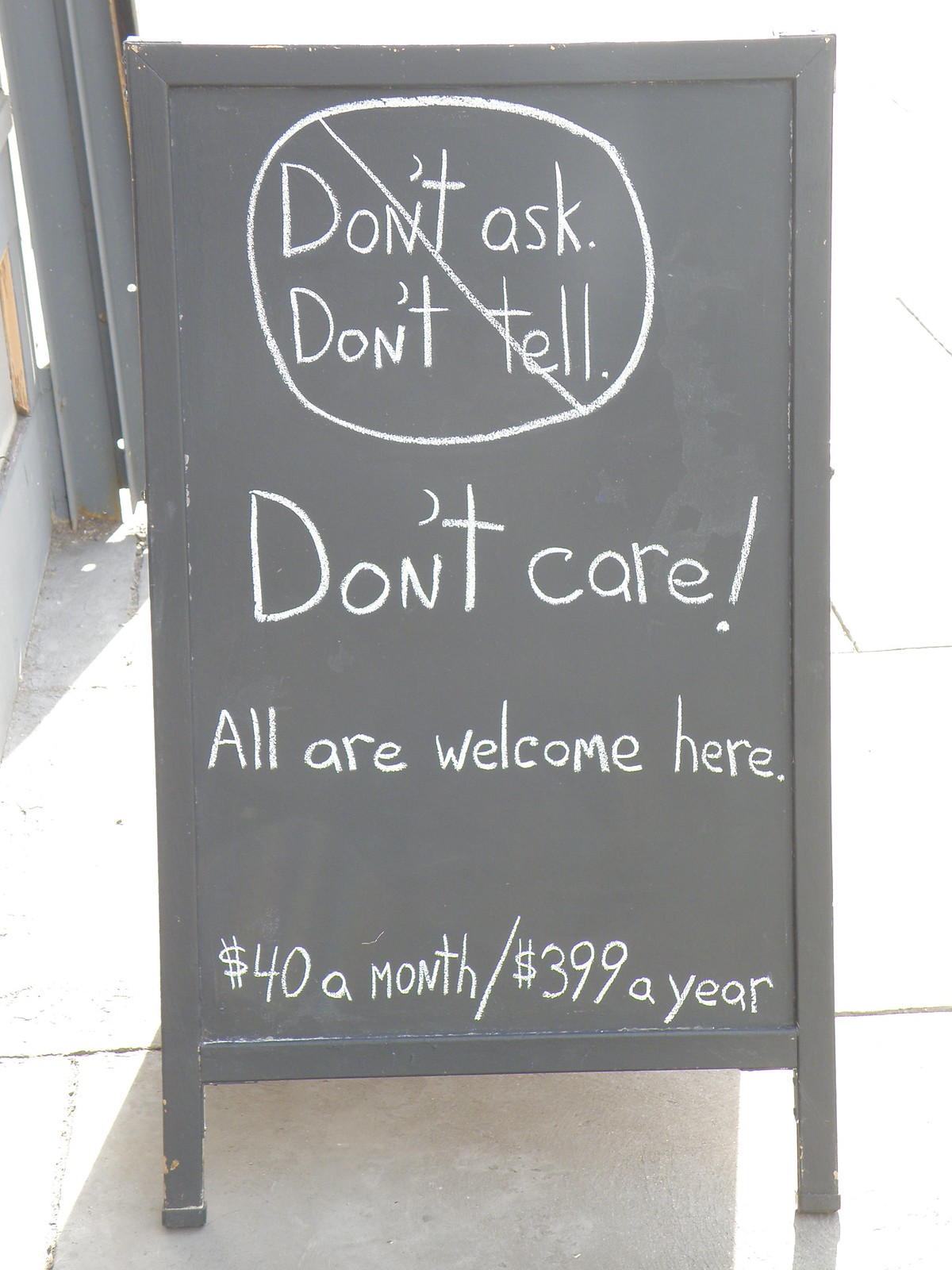The image features a foldable blackboard sign, approximately 2 to 3 feet tall, positioned on a light gray concrete street, suggestive of a business setting. The sign, despite some chipped paint revealing an underlying brown layer, prominently displays text written in white chalk. At the top, the phrase "Don't ask, don't tell" is enclosed in a circle with a slash through it, followed by "Don't care!" Below this, in smaller font, the message reads, "All are welcome here." At the bottom, pricing information is listed: "$40 a month / $399 a year." Two small posts on either side support the centrally placed sign. This scene depicts a welcoming and inclusive message from a business or store.